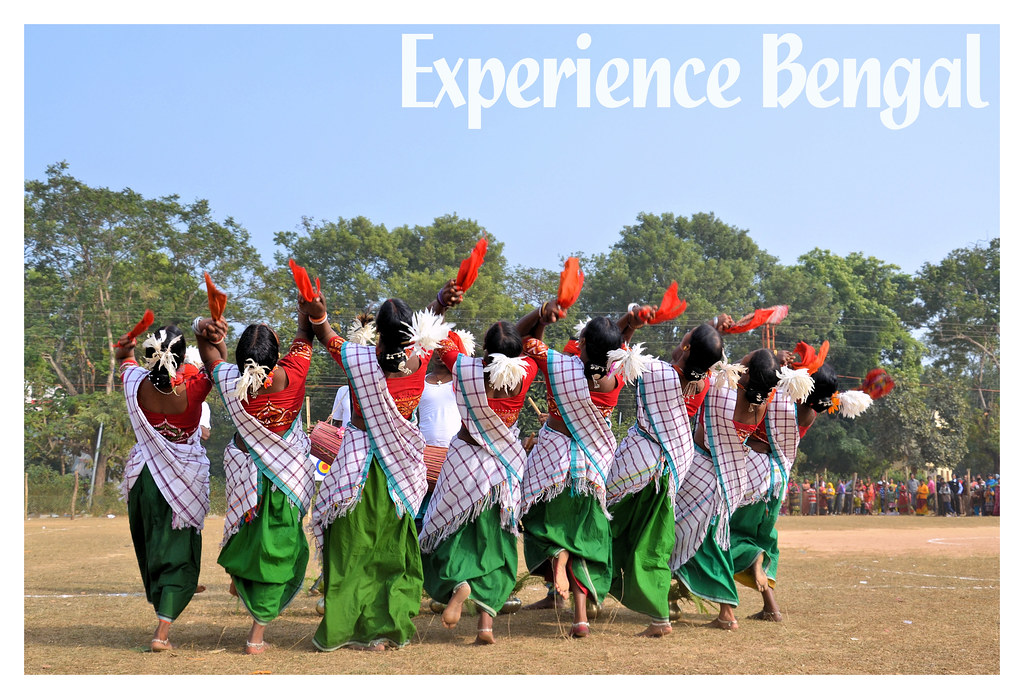The image is an advertisement for Bengal Tourism, prominently featuring the tagline "Experience Bengal" in the upper right corner. It showcases a vivid and detailed depiction of a traditional tribal dance performed by Bengalese villagers in a sunny outdoor setting. The dancers, a group of barefoot women, are adorned in vibrant traditional attire that includes green skirts and orange midriff tops. Additionally, they wear white and blue plaid scarves draped over their shoulders and teal-striped scarves around their waists, complemented by anklets and white feathers intricately styled in their hair adorned with flowers. Each dancer holds orange fans or scarves in their hands, which they raise as part of their synchronized ritualistic dance. In the background, a large crowd of onlookers can be seen, gathered to witness this cultural spectacle, highlighting the immersive, authentic experiences awaiting travelers in Bengal. The scene is framed by a clear blue sky and the tops of surrounding trees, emphasizing the natural beauty of the setting.